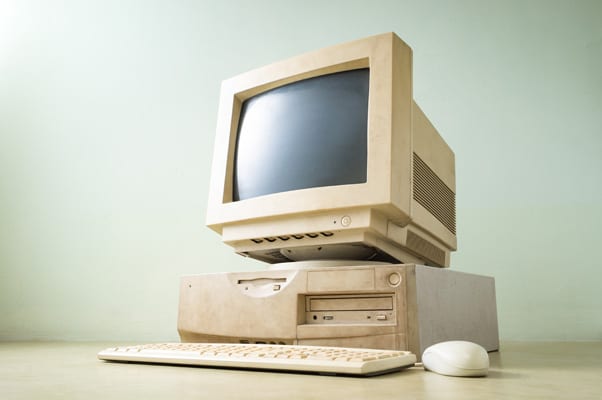The image depicts a vintage computer setup, reminiscent of the early 1980s or 1990s. It is placed on a light-colored table against a solid light grayish-blue wall. The monitor is a bulky, box-shaped unit with a black screen, indicating it is turned off. The top-left corner of the scene is softly illuminated, likely by natural light streaming in from a window. The monitor, which is stained a dingy beige, features various dials for adjusting settings like lighting and contrast, and a floppy disk slot. Just below the monitor, there's the main computer base, which shares the same dirty beige color. On the table in front of the computer, a flat, wired keyboard rests alongside a small white wired mouse. The perspective of the photo suggests it was taken from a low angle, perhaps with the camera positioned on the floor, looking slightly upward at the computer setup.